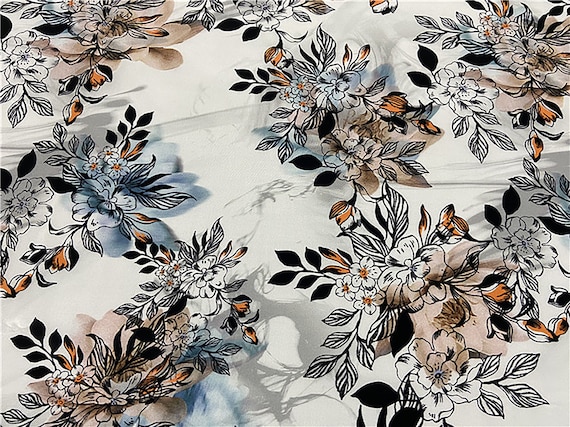This illustration showcases a detailed floral design on an off-white or white background, reminiscent of a watercolor painting or perhaps a tablecloth. It features a variety of flowers, with some appearing as delicate line drawings in black and gray, while others are partially colored. The colored elements include a few black leaves, some burnt orange and tan petals, and vibrant blue flowers. The design is accentuated by swirly lines that mimic the appearance of a water surface, creating a sense of the flowers floating. The flowers are randomly and densely arranged, covering the entire surface. The intricate detailing and the mix of line work with sporadic coloring give the illustration a dynamic and artistic vibe, blending simplicity with splashes of color.